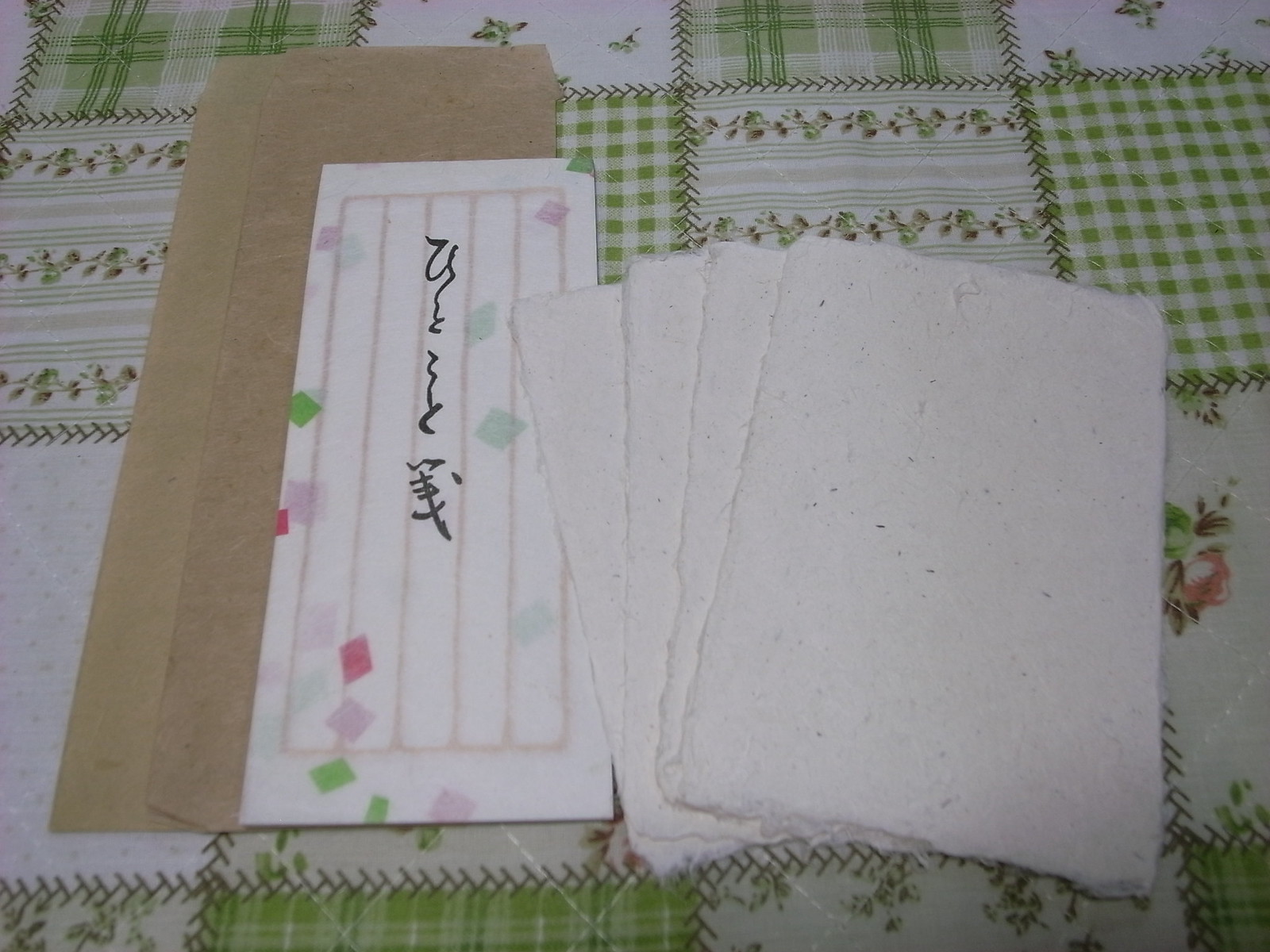The image features a homemade-looking quilt serving as the backdrop. The quilt is meticulously crafted with several squares that highlight a diverse patchwork of light green, white, and hints of pink floral patterns. Among these, some squares are checkered while others showcase floral prints and linear designs, all interwoven with detailed stitching. On the left side of the quilt, a piece of tan material can be seen, and atop this lies an object that appears to be a piece of material with lined and black, possibly foreign, writing. To the right, there are four pieces of thick, white material, likely recycled or homemade paper, fanned out with rough, rugged edges and speckled with flecks, as though compressed from various items. This collection of items, resting on the beautifully stitched quilt, paints a scene filled with a rustic, handcrafted charm.